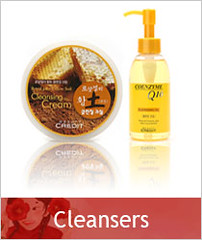The image is an advertisement for a cleanser, presented with a clean white background. At the bottom of the image, there's a prominent red banner with white text that reads "Cleansers." To the left of this banner is an illustrated girl with dark hair, a red flower over her right eye, and another red flower behind her left ear, giving a whimsical and cartoonish feel to the ad. Central to the image are two cleansing products: 

- On the left, there's a cylindrical container labeled "Cleansing Cream," adorned with a honeycomb design. Notably, the container has a reflective surface beneath it that mirrors the image.
- To the right of the container is a transparent yellow bottle, featuring a dark yellow pump and a darker yellow banner around its middle, though the specific details remain indistinct due to the small size and distance.

The overall impression is reminiscent of a product thumbnail one might encounter while shopping on platforms like Amazon, emphasizing both the cleanser's visual appeal and brand identity.